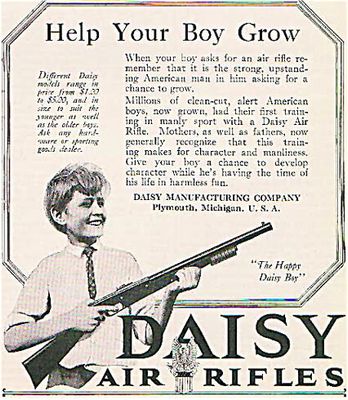This old-fashioned advertisement for DAISY air rifles, set on a beige-colored background with a seven-sided frame-like border at the top, promotes the virtues of buying an air rifle to help boys grow into upstanding American men. The text "Help your boy grow" is prominently displayed beneath the border. It emphasizes that different DAISY models range in price from $120 to $500 and are available in sizes suitable for younger as well as older boys. 

The ad features a black-and-white illustration of a young, smiling Caucasian boy dressed in a button-down white shirt and a small tie, holding a DAISY air rifle and looking towards the right. It appeals to parents by suggesting that when a boy asks for an air rifle, it is the strong, upstanding American man in him seeking a chance to grow. The advertisement highlights that millions of clean-cut, alert American boys, now grown, had their first training in manly sport with a DAISY air rifle, which mothers and fathers now recognize as a means to develop character and manliness. 

The ad concludes by encouraging parents to give their boys a chance to develop character while having harmless fun, with the tagline "The happy DAISY boy" at the bottom, alongside the DAISY Manufacturing Company logo from Plymouth, Michigan, USA.